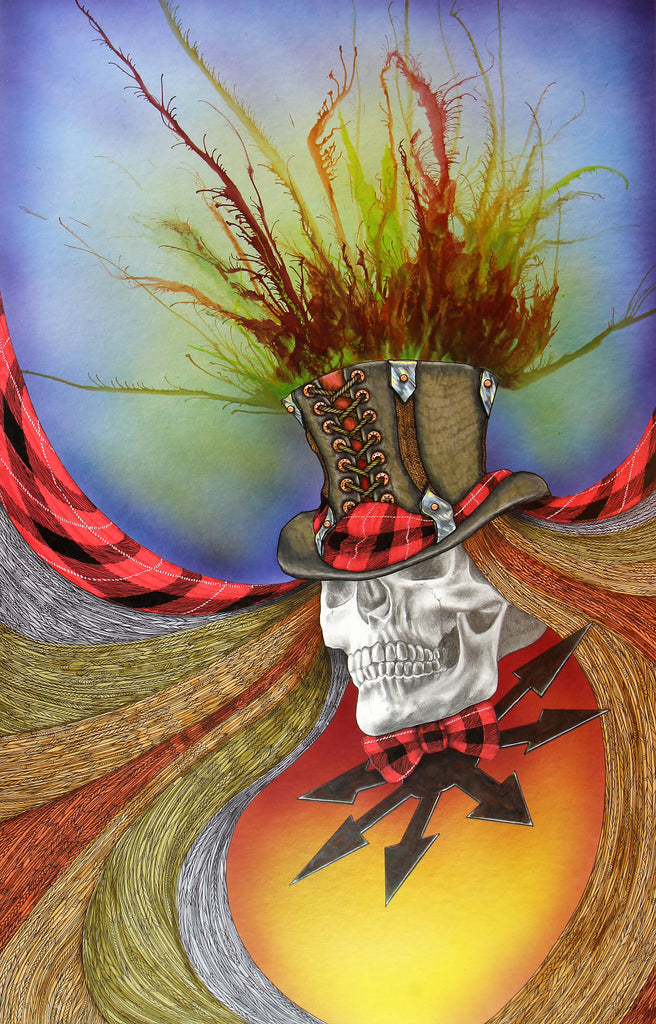This image showcases a detailed, artistic rendition of a skull adorned with a steampunk-themed top hat. The hat is intricately laced up the front with metal hooks and is wrapped with a striking red flannel material, which also forms a bow tie beneath the skull. Emerging from the open top of the hat are various elongated elements resembling feathers or thin twigs in dark reddish-brown, lime green, and blue shades, creating a dynamic and colorful plume. The skull itself is centered in the image, where its base is adorned with a plaid-patterned bow tie and what appears to be a throwing star. Flowing from the sides of the skull is swirling, rainbow-colored hair with hues of oranges, yellows, browns, and greens. The background shifts to a reddish and yellowish-orange gradient, reminiscent of a sunset, enhancing the vivid and surreal atmosphere of the composition.